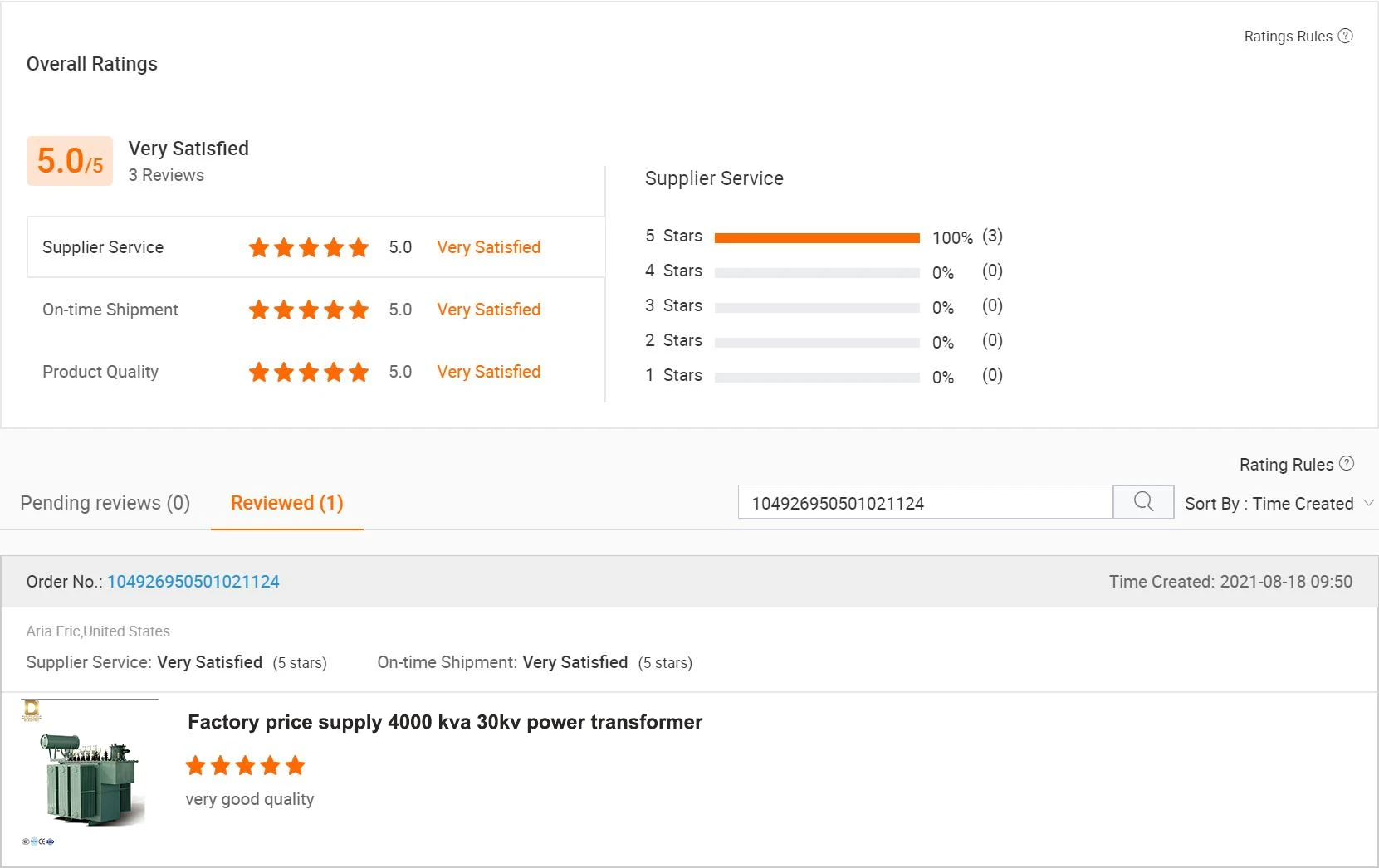This image depicts an online shopping website order summary, predominantly featuring a white background adorned with accents of reddish-orange. All the textual information is rendered in black. The layout is divided into two primary panels: the top panel, occupying about two-thirds of the display, and the bottom panel, making up the remaining one-third.

In the top panel, the focus is on the ratings for an item. The prominent text highlights that the item is rated 5.0 out of 5, accompanied by the phrase "Very satisfied." There are three reviews contributing to this rating. Detailed star ratings are provided: Supplier Service, On-time Shipment, and Product Quality all receive five stars each. To the right, "Supplier Service" is reiterated with a five-star rating, labeled as 100%, with a parenthetical note indicating that three ratings have contributed to this score.

The bottom panel displays the review status of the order, showing "Pending Reviews: 0" and "Reviewed: 1," with "Reviewed" emphasized by an orange font and an underline. To the right, there is a product number and a search bar for ease of navigation. Below, a gray banner labeled "Order Number" precedes a long series of digits, identifying the specific order. The creation date of the order is noted as sometime in 2018.

Further details within the bottom panel include a product description: "Factory price, supply, 4000 kVA, 30 kV power transformer," rated five stars with the review "very good quality" written in lowercase beneath it. A thumbnail image of the transformer, situated on a white background, appears to the left of this text, giving a visual reference to the ordered item.